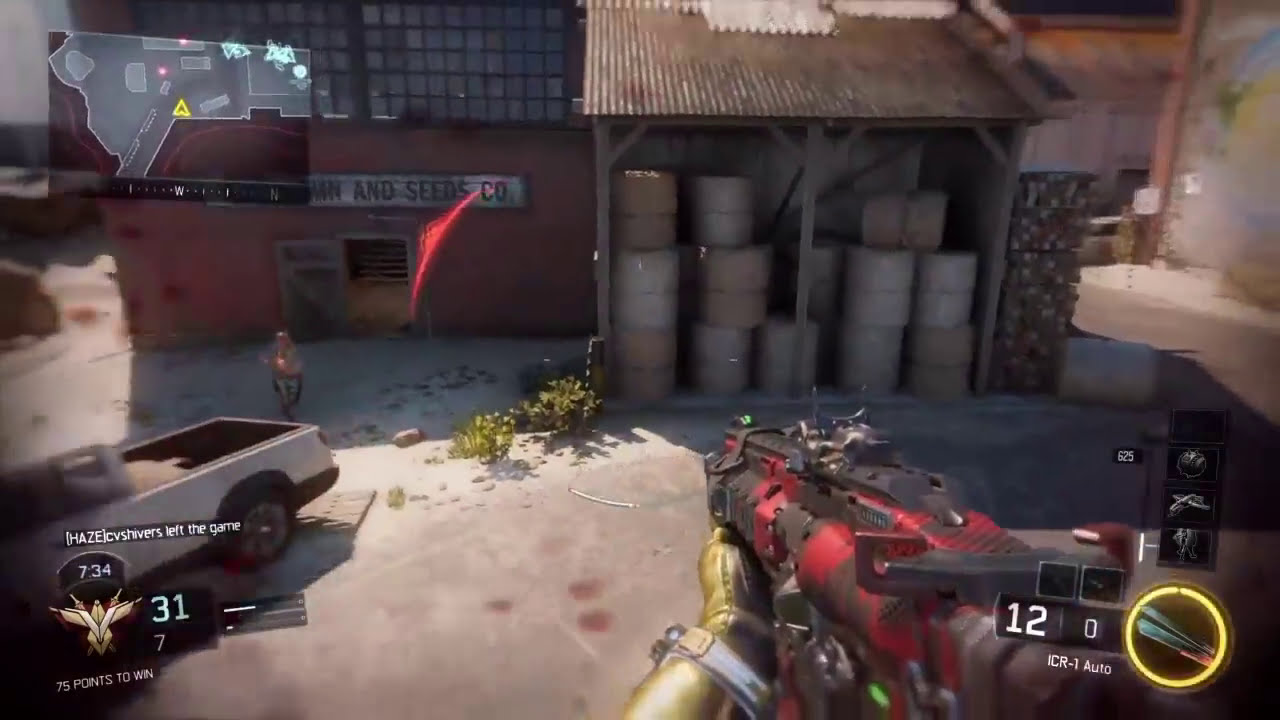In this screenshot from a first-person perspective video game, the player holds a distinctive red and black gun, with a gloved, gold-encased hand visible. The gun interfaces display the numbers "12" and "0," and a label reading "ICR-1 Auto" all on a black background. Additionally, there's a yellow lit-up circle with an object in the middle, potentially representing weaponry, in the bottom right corner. A notification in white letters, stating "Hayes CBS Servers left the game," is also visible. 

In the background, the player appears to be in an outdoor setting with a variety of structures. To the left, there's a red building labeled "Lawn and Seeds Company" with "Co" prominently displayed in dark letters against a white backdrop. Part of another word ending in "MN" is noticeable, cut off from view. Beside this building, an open door reveals stairs, further accentuating the scene's detail. Nearby, a hot shack loaded with barrels or drums, possibly for oil, stands with a brick wall adjacent to it. 

A pickup truck and a vehicle are also present in this scene. The floor and various structural elements exhibit gray, white, tan, and brown tones, including a rusted metal roof and glass windows. A gray map with a yellow triangle marking a specific spot is placed in the top left corner. 

The game interface shows various stats: "734" near a winged creature resembling a bug, with additional numbers "31," "7," and an objective of "75 points to win." A humanoid figure approaches the player, seemingly running while wielding a gun. The overall image quality appears somewhat rough-edged and blurry, capturing the chaos and action typical of intense gaming moments.